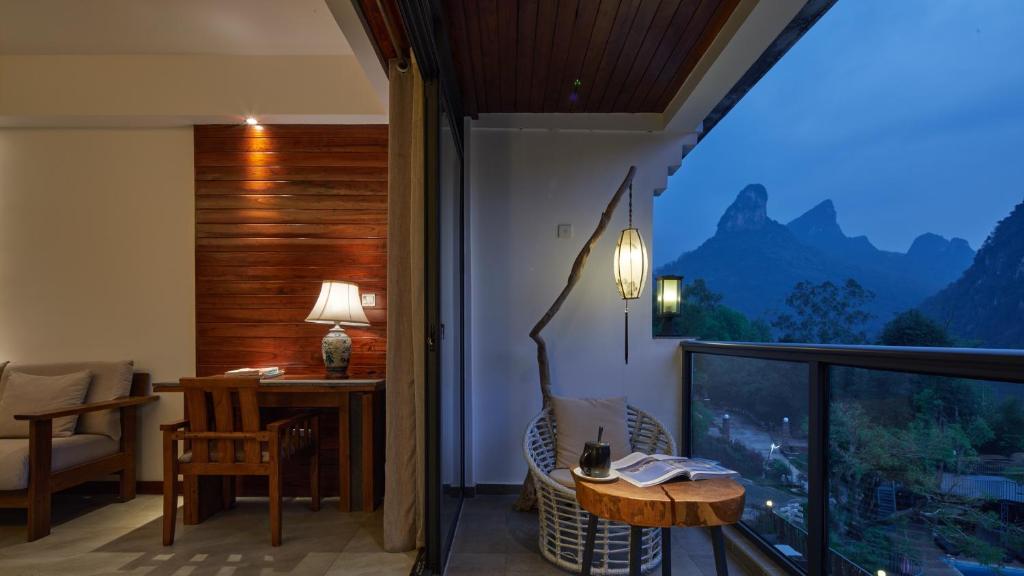The image depicts a cozy, indoor-outdoor living space transitioning from a warm, inviting room to a scenic balcony. On the left side of the photograph is the interior, furnished with a dark mahogany wooden desk and matching chair, a small ceramic lamp with an off-yellow lampshade casting a soft glow, and a hint of a light gray cushioned futon partially cropped out of the frame. The walls feature dark brown wooden panels complemented by a cream-colored section. A carpet covers the floor, adding to the room's warmth.

Transitioning to the right side, the scene opens onto a clear-glass balcony. A small, round wooden coffee table holds a black mug and a book or magazine, suggesting a peaceful, leisurely setting. A white wicker chair with a light brown pillow is positioned nearby. Above, a unique wooden lighting fixture hangs down, casting a gentle yellow light.

Outside, the view extends over a handrail to a twilight scene of darkening blue skies, a distant mountain range, and lush green trees below. The image captures the serene beauty of the surrounding nature, with a potential small walkway visible in the distance, emphasizing the elevated perspective of a high-floor balcony in a house or apartment.